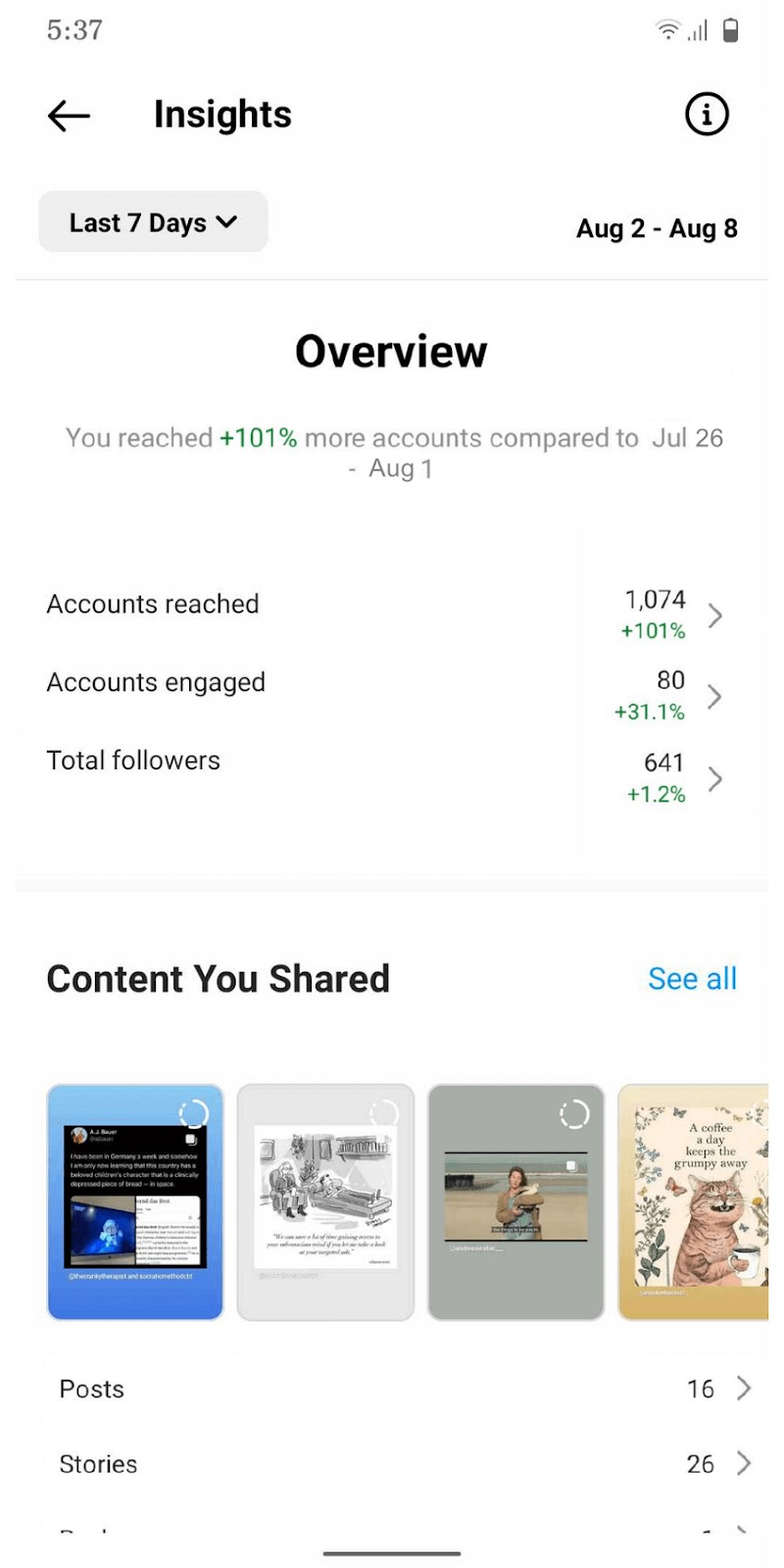The image depicts a detailed overview of a cell phone screen, specifically displaying social media insights. In the upper left corner, the screen shows the time, "5:37." In the upper right corner, the screen displays icons for Wi-Fi signal strength, cellular connection, and battery status, which is at half capacity.

Below these icons, a navigation bar features a left arrow labeled "Insights" and, on the right side, an eye within a circle icon. Underneath this bar, the text reads "Last 7 Days" with a drop-down option, and to the right, the date range "August 2 - August 8" is displayed.

A horizontal line separates these sections from a summary text that reads "You have reached +101% more accounts compared to July 26 - August 1," with the "+101%" in green and the rest of the text in grey. Under this summary, metrics are outlined:

1. **Accounts Reached**: "1,074" with an indication of "+101%", and a right arrow.
2. **Accounts Engaged**: "80" with a "+31.1%" increase, and a right arrow.
3. **Total Followers**: "641" with a "+1.2%" increase, and a right arrow.

All percentage values are highlighted in green, while the other text is in black or grey. 

A grey line under these metrics separates them from the "Content You Shared" section, which appears on the left side. "See All" is on the right in teal color. Below this text are four square thumbnails representing posts, where the last square is partially cut off, suggesting a carousel format for additional posts. 

At the bottom, "Posts: 16" is indicated on the right side, with a right arrow next to it.